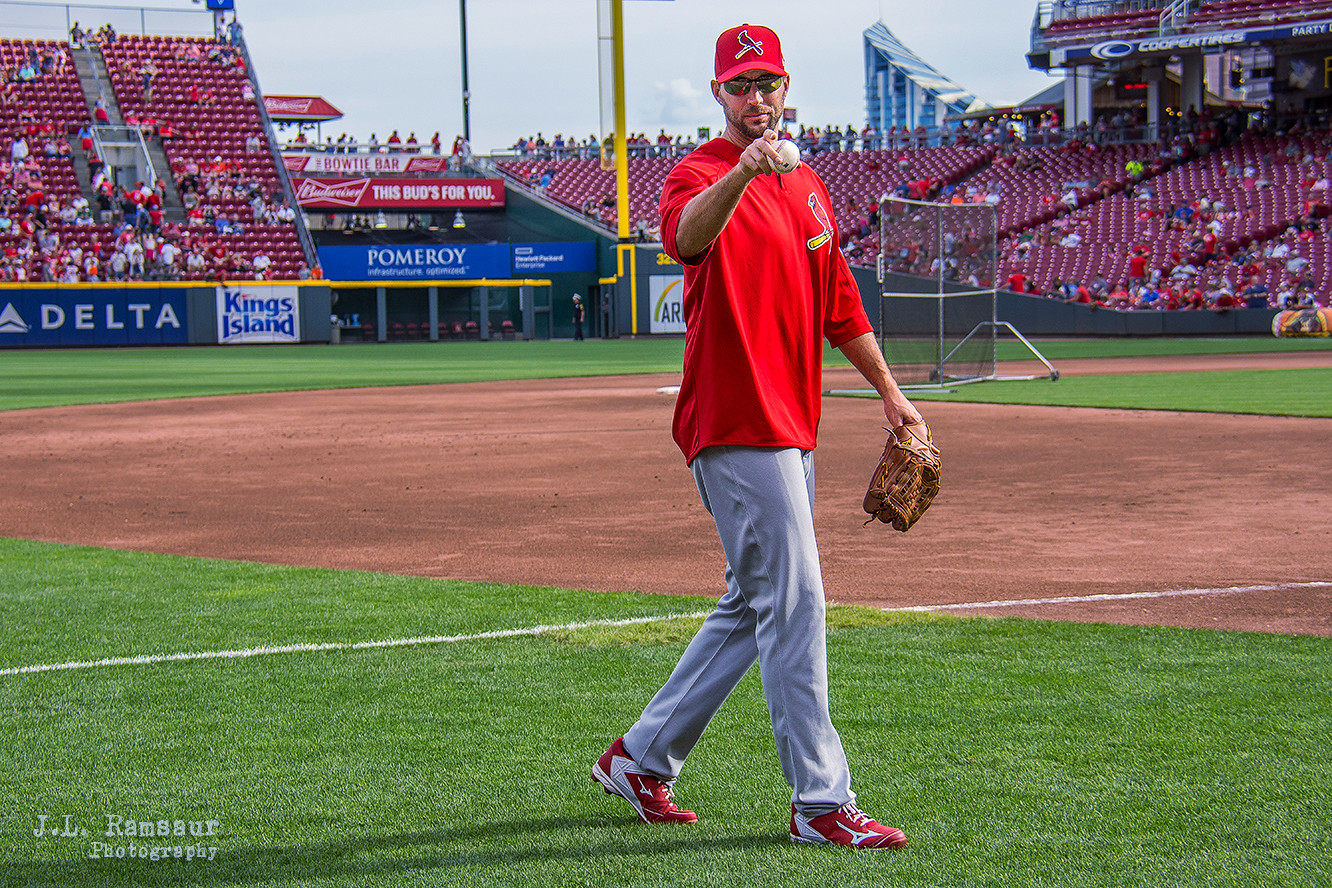The photograph captures a moment on a baseball field, with sandy brown dirt and short artificial green grass marking the different areas of play. In the bottom left corner, the watermark "J.L. Ramser Photography" in slightly transparent white text is visible. Dominating the foreground and center of the image is a man outfitted in a St. Louis Cardinals uniform. He is walking towards the right, wearing bright red shoes with white stripes and soles, gray pants, and a red graphic t-shirt emblazoned with a red bird perched on a yellow bat. 

He is pointing towards the camera with a baseball in his right hand, suggesting he might be about to toss it to a fan. His baseball glove is loosely fitted on his left hand. Given the sparse crowd in the background stands, it appears to be a pre-game moment, possibly during batting practice. There is a protective metal cage in front, likely to shield players taking grounders from flying balls. The background reveals a cloudy sky, the outfield, and a yellow foul pole. The subtle interaction between the player and the scattering of fans, along with the casual setting, suggests an informal or practice scenario rather than an ongoing game.